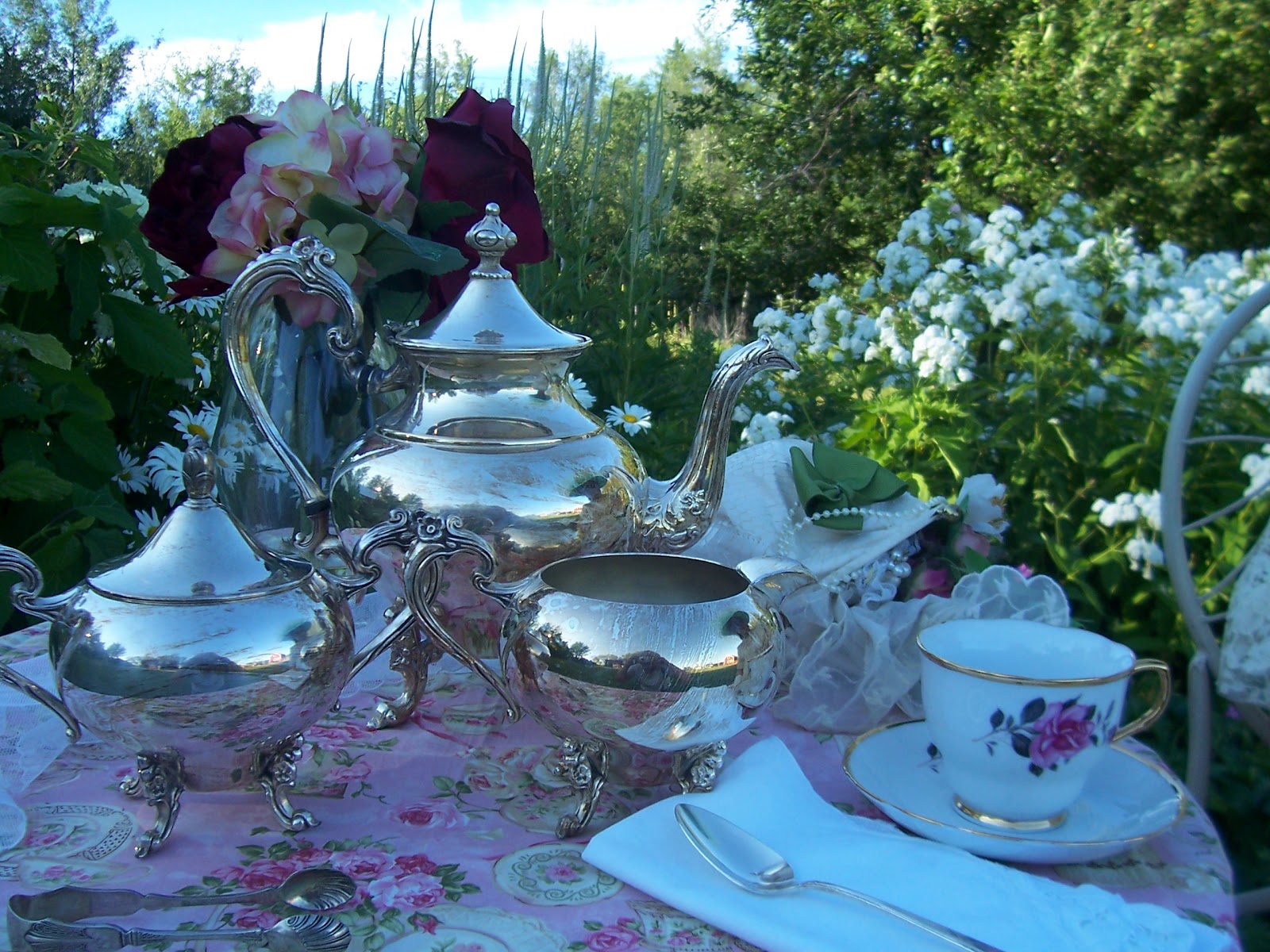This photograph captures an exquisitely detailed outdoor tea party set in a lush garden surrounded by trees and vibrant flowering bushes. The setting features a table adorned with a multicolored, ornate tablecloth showcasing purple, pink, and green floral patterns that harmonize beautifully with the garden's greenery and abundant blooms. A refined collection of tea-serving pieces, including a large, footed silver teapot, a lidded sugar container, and a creamer pitcher, are the focal points, exuding an elegant, English-style charm. A single china teacup with gold trimming and a delicate pink floral design sits next to a white cloth napkin, topped with one of three silver spoons scattered strategically across the tablecloth. Complementing the arrangement is a vase brimming with a mix of large, lush flowers in wine, white, and lavender hues, adding a burst of color and life to the scene. The garden ambiance is enhanced by the sunny day, with blue skies and fluffy white clouds peeking through the leafy canopy, creating a picturesque backdrop for this charming al fresco tea gathering.